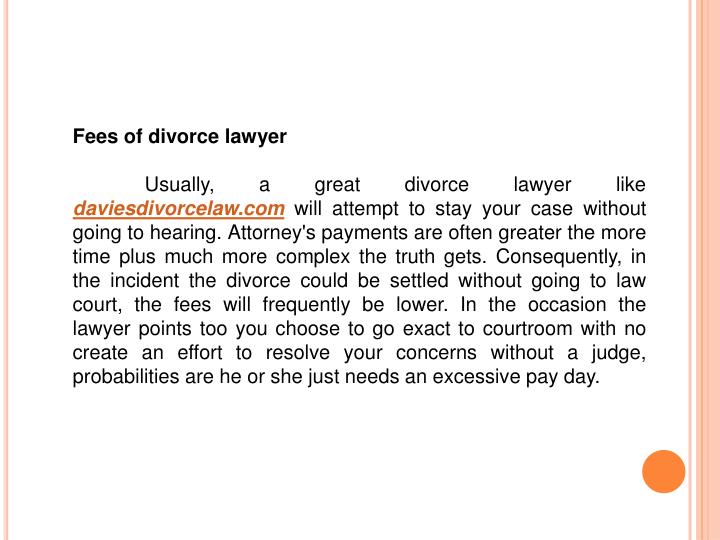The image is an infographic designed to advertise divorce lawyer services, featuring only text on a white background. It is framed with a distinctive pink border on the left and a thicker, multi-lined pink border on the right, culminating in an orange circle at the bottom right corner. The text is well-centered and predominantly black, resembling typewriter font, with key highlights in orange. The title at the top, "Fees of Divorce Lawyer," is in bold, followed by a paragraph detailing that a reputable divorce attorney, referenced as DaviesDivorceLaw.com (hyperlinked in orange), typically seeks to settle the case without court hearings, thus keeping fees lower. If the case proceeds to court without attempts at resolution, it suggests the lawyer may be seeking higher compensation. This infographic appears intended for a website to promote the advertised divorce services.